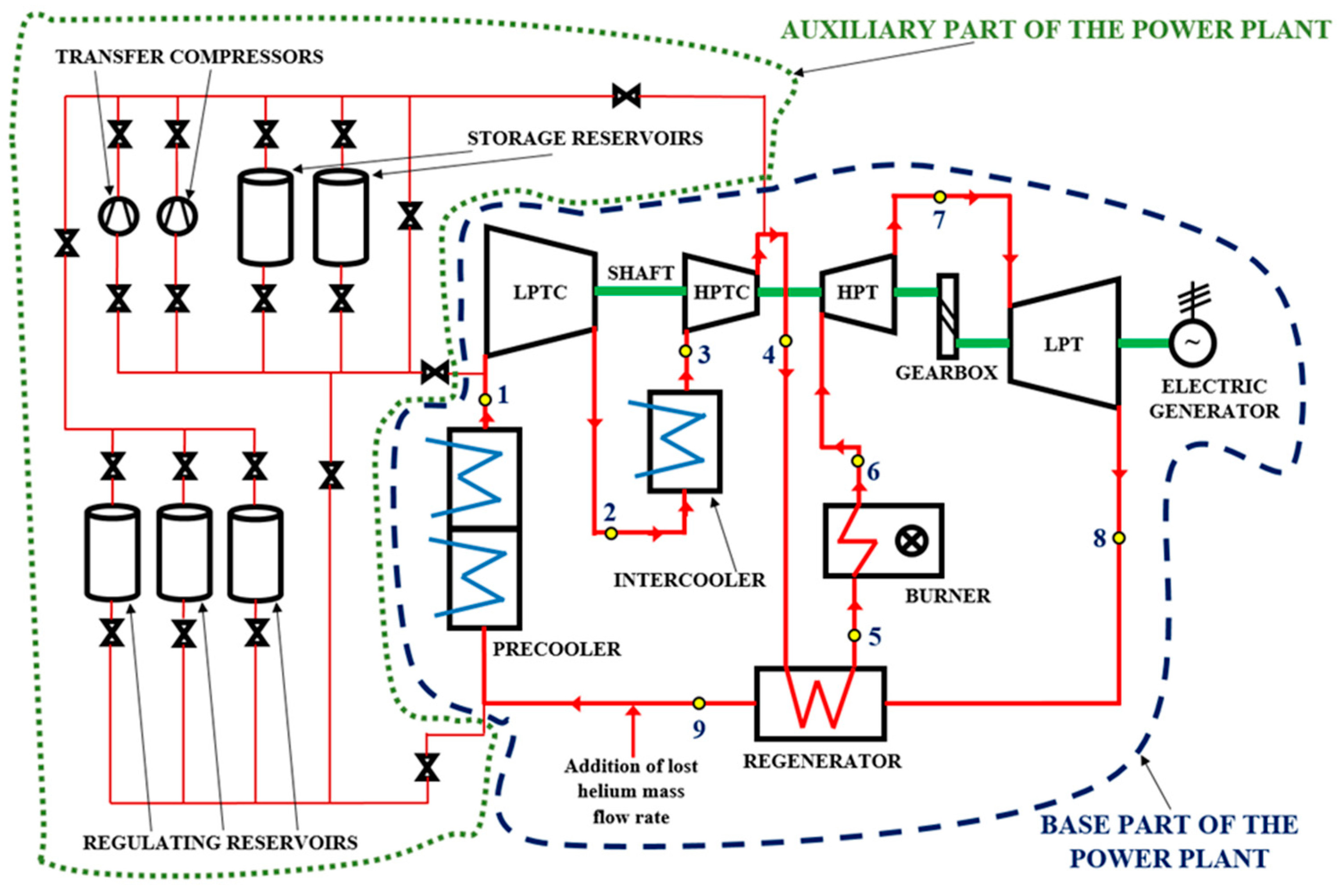The diagram is a detailed and colorful depiction of a power plant, encompassing numerous components and sections distinguished by varying colors and annotations. On the bottom right, the "BASE PART OF THE POWER PLANT" is highlighted within a navy blue dotted line, and the top right section, designated as the "AUXILIARY PART OF THE POWER PLANT," is marked with a green dotted line. Most of the text is in bold, capitalized Times New Roman font, except for one label in the bottom middle— "addition of lost helium mass flow rate," which is uncapitalized.

The diagram features various interconnected parts, such as transfer compressors, storage reservoirs, regulating reservoirs, pre-cooler, intercooler, burner, regenerator, gearbox, shafts (LPTC shaft, HPTC, HPT, LPT), and an electric generator. These components are linked by red flow arrows, illustrating the operational flow within the power plant. The layout contains symbols and annotations spread throughout, presenting a comprehensive and intricate overview designed to educate viewers about the different parts and their functions within the power plant. The colors displayed in the chart include blue, black, red, and green, making the diagram visually complex and informative.